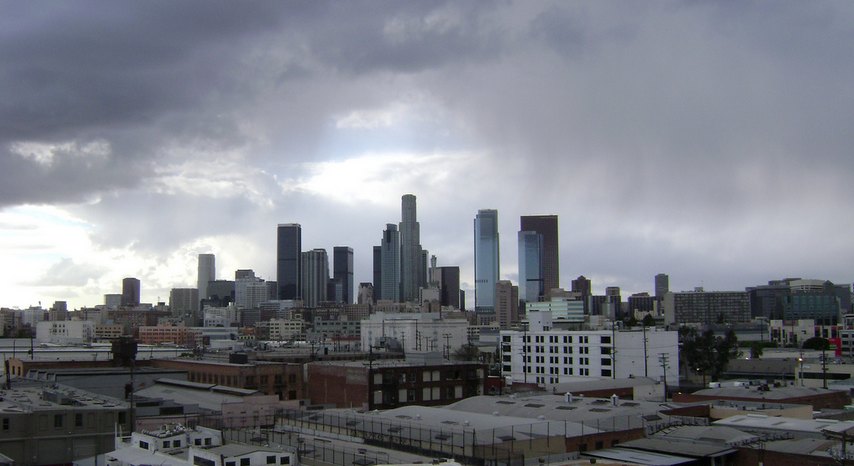The image depicts a faraway view of a cityscape, dominated by a cluster of skyscrapers and high-rise buildings in the background. These towering structures, mostly dark gray and bluish in color, are set against a backdrop of a dim, cloudy sky, suggesting either an early dawn or late dusk setting. The overcast weather casts muted natural light, adding to the gray tones prevalent throughout the scene.

In contrast to the distant skyline, the foreground features more residential elements. Here, there's a mix of low-rise buildings with varying architectural styles; some are one-story structures, and others rise up to three stories. The buildings closer to the viewer display a palette of brown, black, and white, distinguishing them from the more monochromatic, industrial-looking high-rises in the distance.

Of particular note is a white building in the foreground, characterized by rows of dark windows. This structure sits alongside other lighter and darker buildings, creating a clear division between the residential and the taller, business-oriented skyscrapers in the background. The overall grayness and industrial atmosphere of the scene are punctuated by a lighter patch in the clouds where they meet the horizon, offering a slight contrast in an otherwise muted, urban landscape.